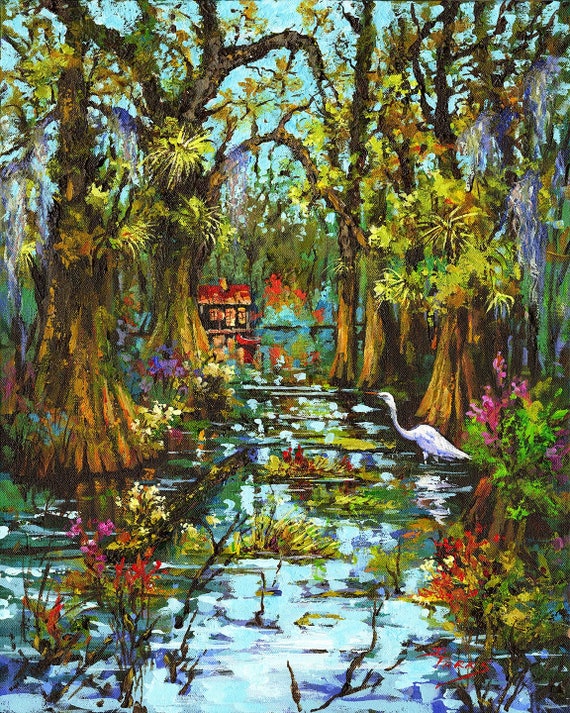The painting depicts a serene forest scene with an abundance of flora and fauna, dominating in a vertical rectangular frame. At the center of the composition runs a river, weaving its way through the landscape, flanked by various plants, flowers, and occasional sticks reaching out of the water. The banks on either side exhibit lush grass and colorful flowers, including white, red, and purple varieties, intermixed with weeds and tall trees. These trees have wide trunks that stretch upward and display a palette of greens, yellows, and browns, reminiscent of weeping willows.

To the left of the center, partially hidden among the foliage, stands a house with a red roof and wooden sides. The house exudes warmth with its glowing windows, suggesting an inviting interior light. In the foreground, a stately crane-like bird, white with a long neck and orange beak, strides through the water with its legs submerged, adding a touch of life to the tranquil scene.

Adding to the natural beauty, the background features a landscape where the forest canopy almost entirely obscures the sky, which peeks through in light blue hues. The body of water reflecting the environment, filled with patches of vegetation, extends from the bottom of the frame to the distant house. The scene is rich with intricate details, from the reflections on the water to the vibrant interplay of colors and textures across the elements within the forest.